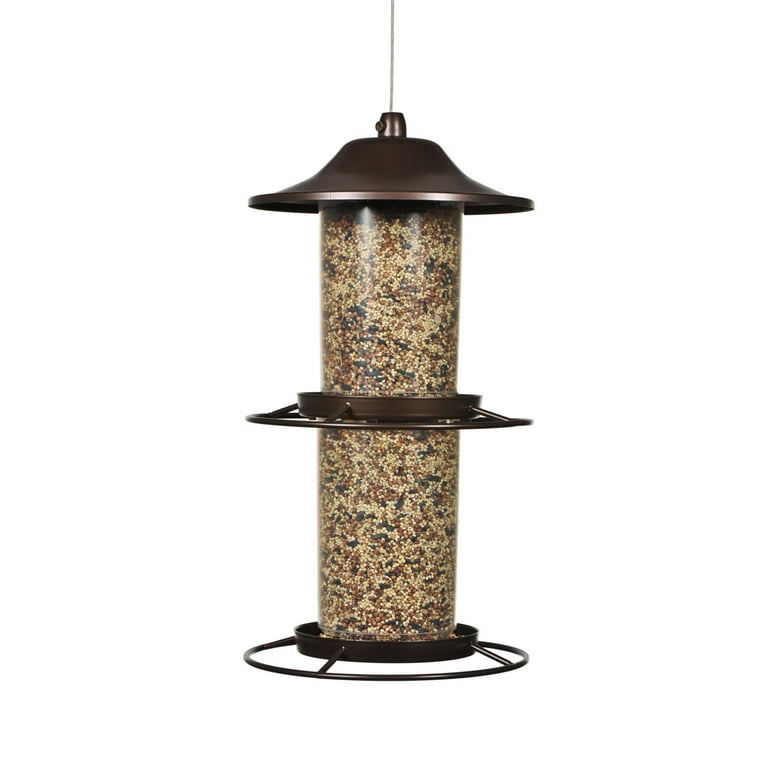The image showcases a large two-tiered bird feeder designed to be suspended in the air by a string or rope attached at the top. The feeder's top section resembles a bell-shaped, brown metal lid that extends outward, likely to deter squirrels and shield the seeds from rain, much like a protective hat. The main body of the feeder is transparent, allowing the viewer to see the mix of multicolored seeds—tan, brown, black, and white—contained within. Each tier includes a small dish in the midsection and bottom to catch and hold the seeds, and features circular footholds resembling a hula hoop for birds to rest on while feeding. The background of the photo is plain white, offering a clean, uncluttered view of the intricately designed feeder.